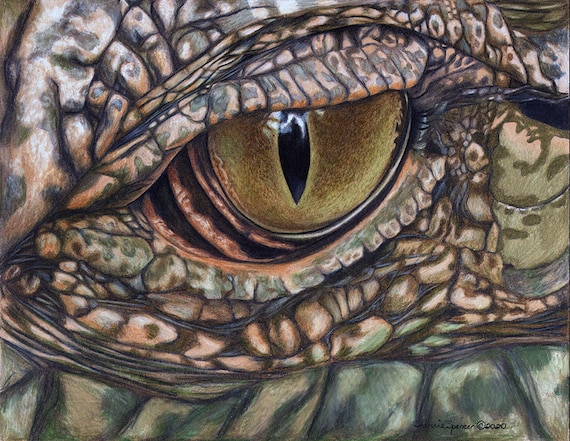This highly detailed image, possibly a digital creation or an exceptionally realistic photograph, features a reptilian creature, focusing primarily on its striking eye. The eye, characterized by a distinctive, pointy oval pupil typical of reptiles, exhibits a cloudy green hue around the center. Surrounding the eye are meticulously rendered scales, which add to the lifelike appearance of the creature. The eyelid, slightly closed, conveys an intense, almost menacing expression. Beneath the eye, intricate details continue to enhance the realism, with subtle shading and texture. In the bottom right corner of the image, a faint signature is visible, hinting at the artist's personal touch.